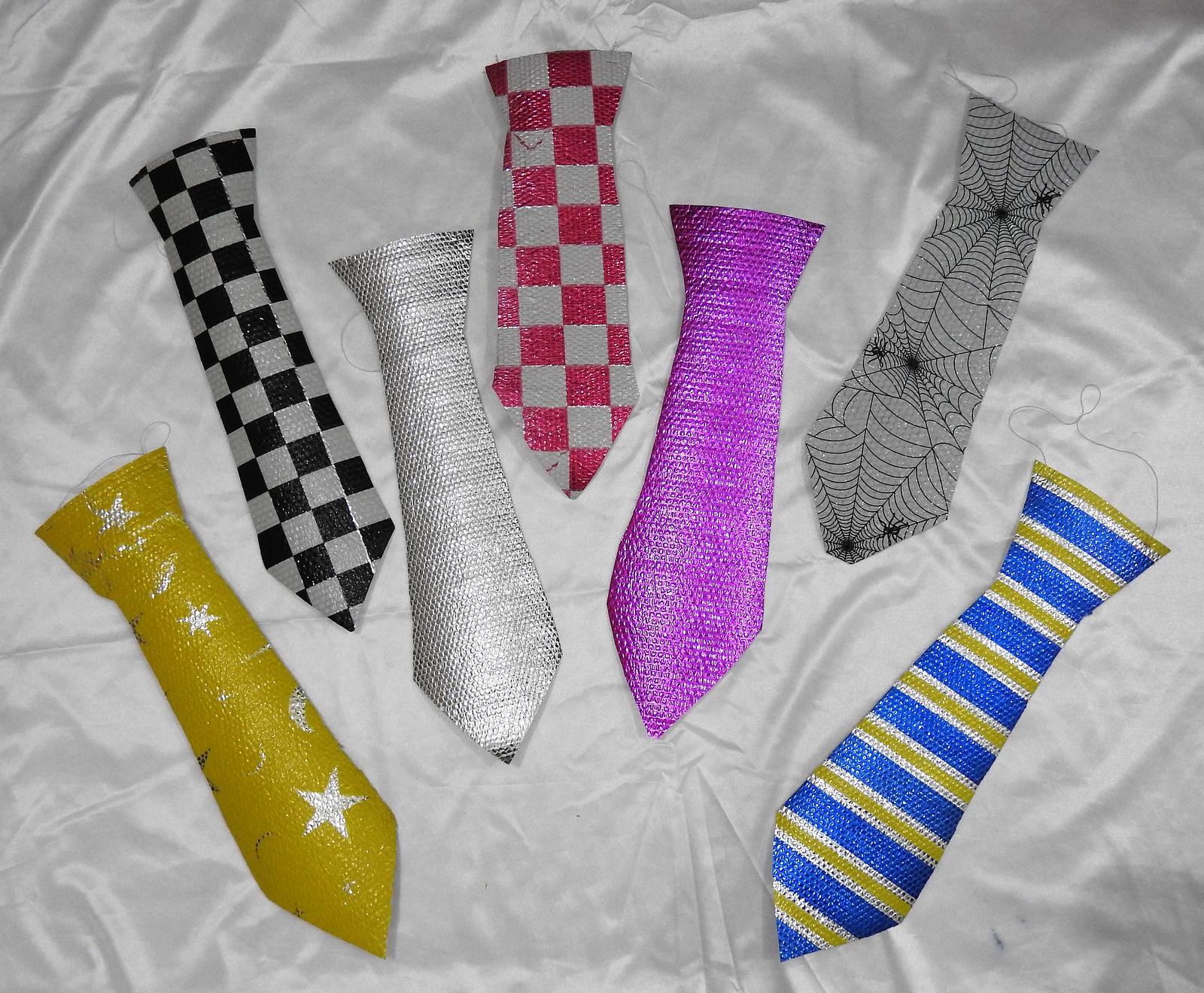This image showcases a collection of seven festive, party-themed ties laid out on a silky, white or gray fabric backdrop. Each tie is fastened with a clear, delicate string designed to be worn around the neck, indicating that they are more for decorative or costume purposes rather than for traditional use. 

From left to right: 
1. The first tie features a vibrant yellow hue adorned with silver stars.
2. Next is a sophisticated black and white checker pattern.
3. The third tie glistens in silver.
4. Following that is a playful red and white checker design.
5. The fifth tie stands out with its rich purple color.
6. The sixth tie is silver embellished with black spiderwebs, adding a touch of whimsy.
7. The final tie alternates between green, silver, and blue stripes, creating a dynamic, festive look.

Together, these ties create a colorful and eye-catching display, perfect for any celebration.